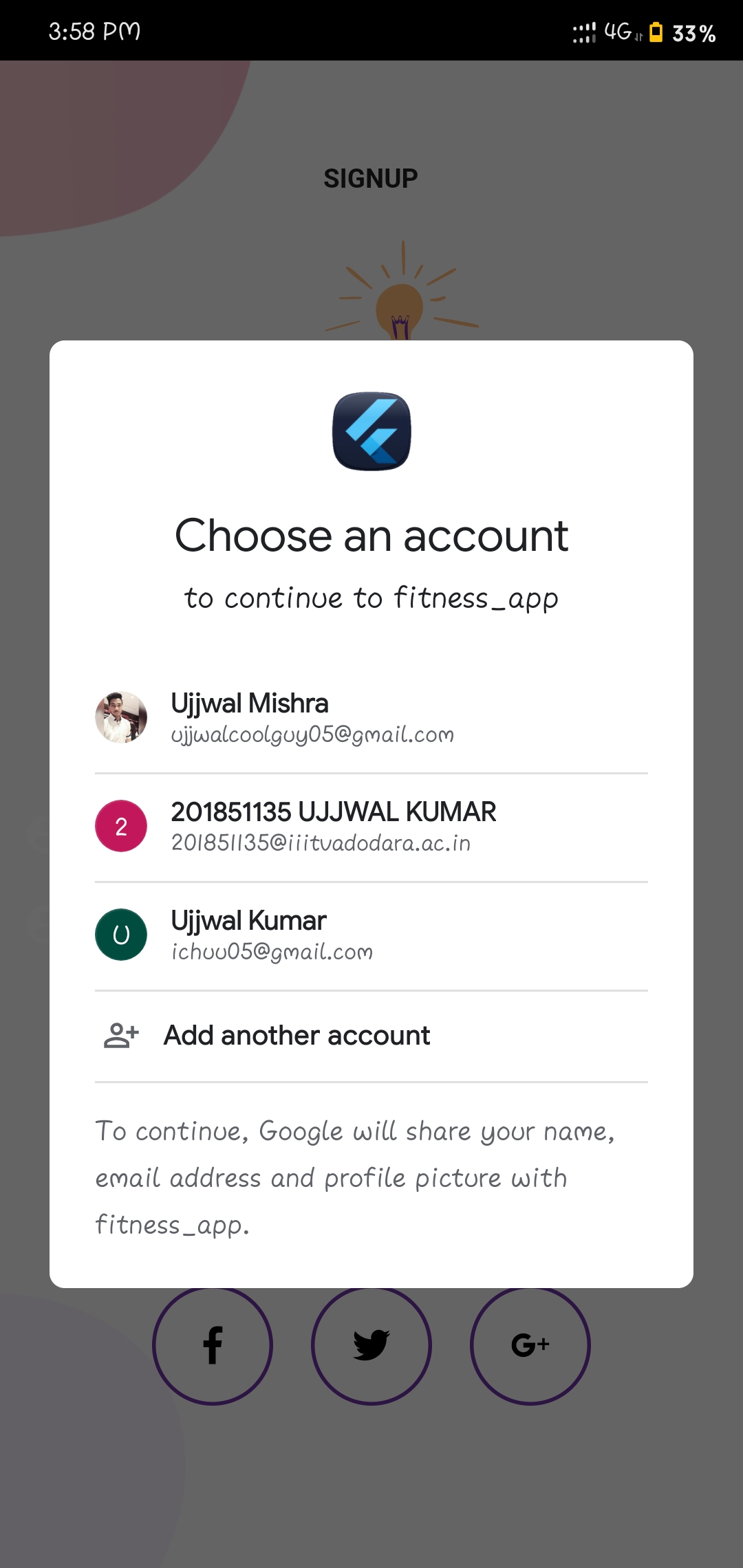The image captures a screen from a mobile device showcasing a sign-up interface for the "Fitness App." The background is slightly grayed out, emphasizing the white pop-up window at the center. A pastel pink curved design adorns the top-left corner of the screen, providing a subtle splash of color.

In the pop-up window, positioned centrally, there's a gray and blue logo at the top, followed by a prompt in black text: "Choose an account to continue to fitness_app." Below this prompt, three different account names are listed vertically. Underneath the third account name, there's a plus icon next to the text "Add another account."

Towards the bottom of the window, smaller text informs the user about data sharing: "To continue, Google will share your name, email address, and profile picture with fitness_app."